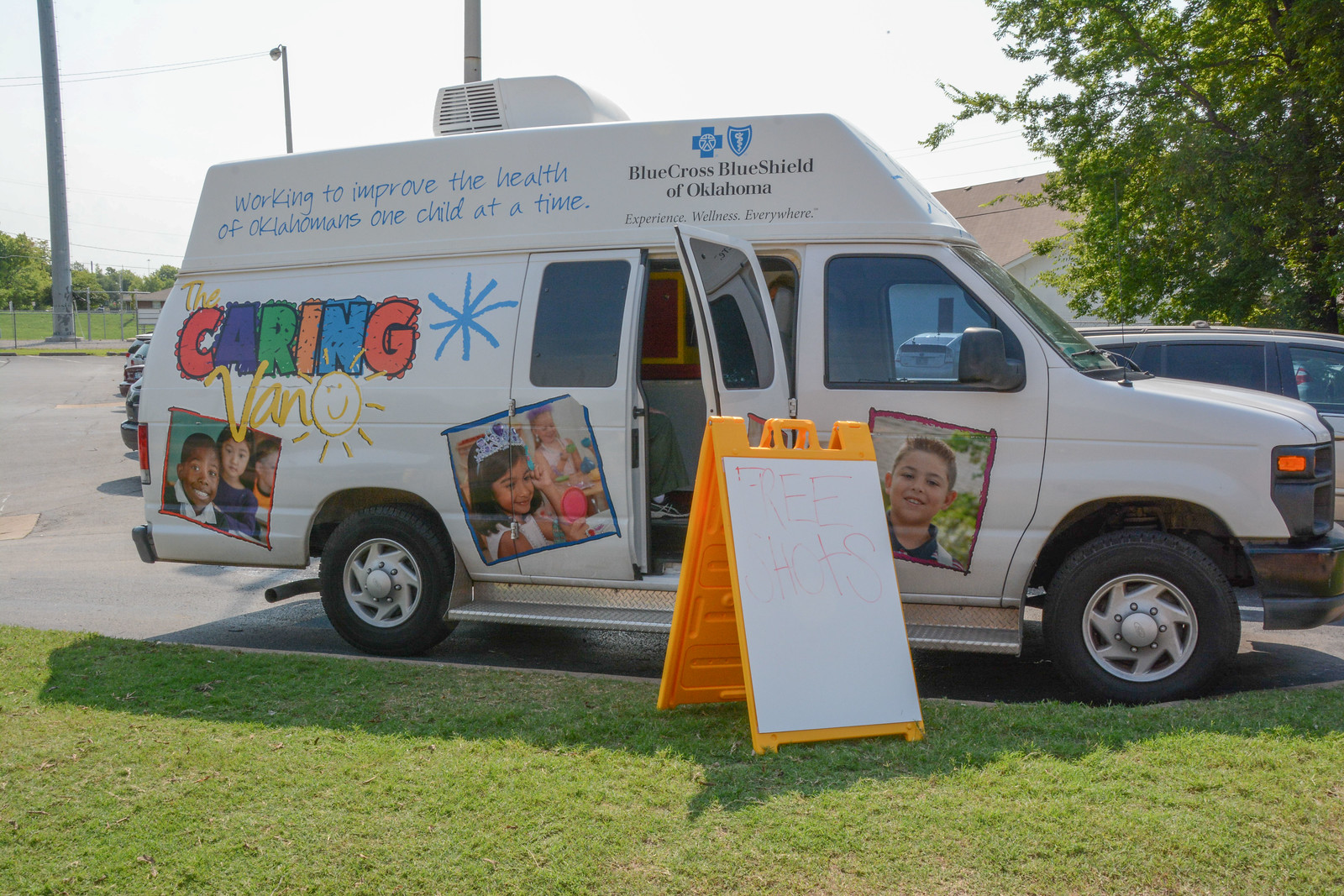The image showcases a white van parked in a lot, surrounded by grass, a building, and trees. The van prominently features Blue Cross Blue Shield of Oklahoma logos and bears the message, "Working to improve the health of Oklahomans one child at a time" at the top. The side of the van is adorned with vibrant, childlike lettering spelling out "The Caring Van," with each letter in a different color—C is red, A is purple, R is green, I is orange, N is blue, and G is orangish-red. Artistically drawn suns and star or firework patterns add a whimsical touch. There are also three clear photographs of smiling children, reinforcing the message of caring and wellness. A yellow setup with a whiteboard displaying the words "Free Shots" in red is placed outside the open side doors of the van, and it features a roof-mounted A.C. unit to accommodate standing visitors inside. The overall impression is one of a mobile unit dedicated to children's health and wellbeing, operating as part of a broader community initiative.